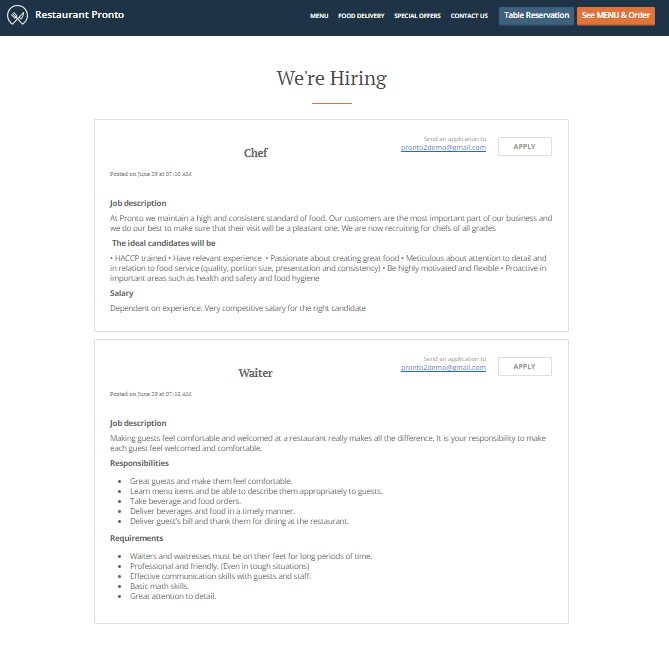The webpage for Restaurant Pronto features a sleek design with a navy blue ribbon across the top. On the left-hand corner of this ribbon, the restaurant's name, "Restaurant Pronto," is displayed in simple white text alongside their logo—a white circle open at the bottom with lines connecting to a crisscrossed fork and knife within the circle.

To the right of the logo, the navy blue ribbon presents various navigation options in white text: Menu, Food Delivery, Special Offers, and Contact Us. Toward the end of the ribbon are two buttons: a blue "Table Reservation" button followed by an orange "See Menu and Order" button.

The central section of the page has a clean white background. At the top, in large navy blue text, are the words "We're Hiring," underlined by a short dark orange line. Below this announcement are two rectangular boxes, each highlighting a different open position.

The first, smaller box, features a Chef position. The word "Chef" is prominently displayed in navy blue text in the center. On the far right of this box, there is a white "Apply" button with navy blue text and a gray border. Below "Chef," in tiny blue letters on the left-hand side, it states "Posted on June 29th at 7:10 AM." Following this, a bold navy blue "Job Description" heading introduces the description text in gray, detailing Pronto's dedication to maintaining high and consistent food standards and the importance of customer satisfaction. The text goes on to invite applications from chefs of all grades and provides further details about the ideal candidate and salary.

The second, longer box details a Waiter position, maintaining the same layout. It includes the posting date and time, a job description, and details about responsibilities and requirements.

This detailed layout underscores Restaurant Pronto's professional approach to recruitment, ensuring potential applicants have all the necessary information presented clearly and concisely.